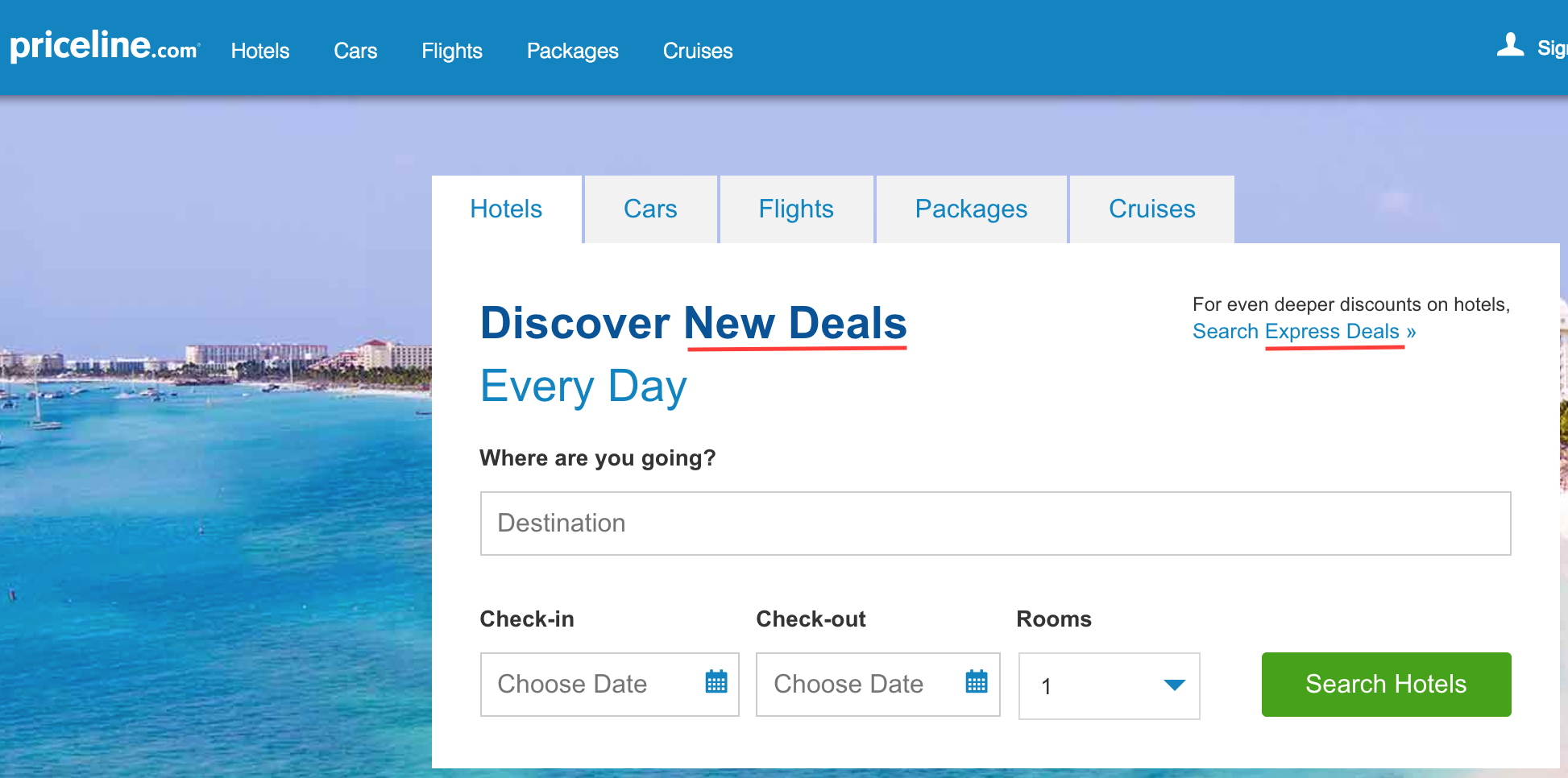**Descriptive Caption:**

The displayed image is a screenshot of a website. At the top of the page, there is a prominent ocean blue banner with the text "Pricevine.com" in white. The word "Pricevine" is in a thicker, larger font, while ".com" is in a smaller, finer print. Just below the banner, there is a navigation menu with the categories "Hotels," "Cars," "Flights," "Packages," and "Cruises," each with an uppercase initial letter.

On the right side of the header, there is an icon that appears to be a silhouette of a person's head and shoulders. Beside the icon, partially cut-off text reads "S-I-N."

The main background of the webpage features a serene scene with a purplish-blue sky and purple-tinted clouds. Below this sky area, an idyllic coastal view is visible, including a beach lined with trees, a body of water resembling the ocean, and several boats floating on the surface.

A prominent white pop-up covers part of this background. The pop-up header repeats the navigation categories: "Hotels," "Cars," "Flights," "Packages," and "Cruises" in blue text. Below the header, it says "Discover New Deals," with "New Deals" underlined in red. Further down, text prompts read "Every Day," "Where Are You Going," "Destination," "Check In," "Choose Date," "Check Out," "Choose Date," and "Rooms." The "Rooms" field is pre-filled with the number one and includes a drop-down menu for selection. At the bottom of the pop-up, there is a green rectangular button with the text "Search Hotels" in white. 

Overall, this website interface appears user-friendly and visually appealing, designed to help users search for travel deals efficiently.